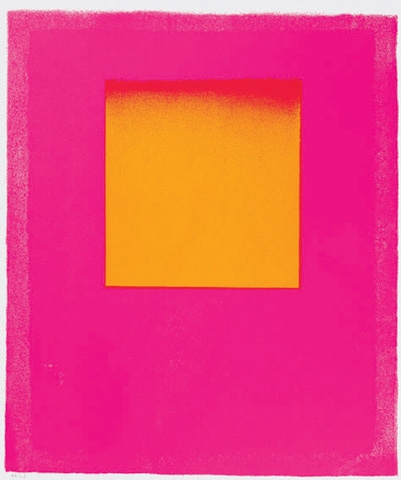This abstract painting on a portrait-oriented canvas features a vivid bright pink rectangle filling the majority of the background. There is a narrow perimeter of light gray, almost white, along the edges, with the top border being slightly wider than the others. Within the pink background, a square shape is positioned slightly above the center. This square is predominantly yellow but transitions into a reddish-orange hue at the top. The colors blend together smoothly, with specks of red extending into the yellow area, creating a dotted effect. The painting has no visible signature or writing. The composition of colors—white, hot pink, yellow, and reddish-orange—adds to the vibrant and dynamic nature of this piece of art.